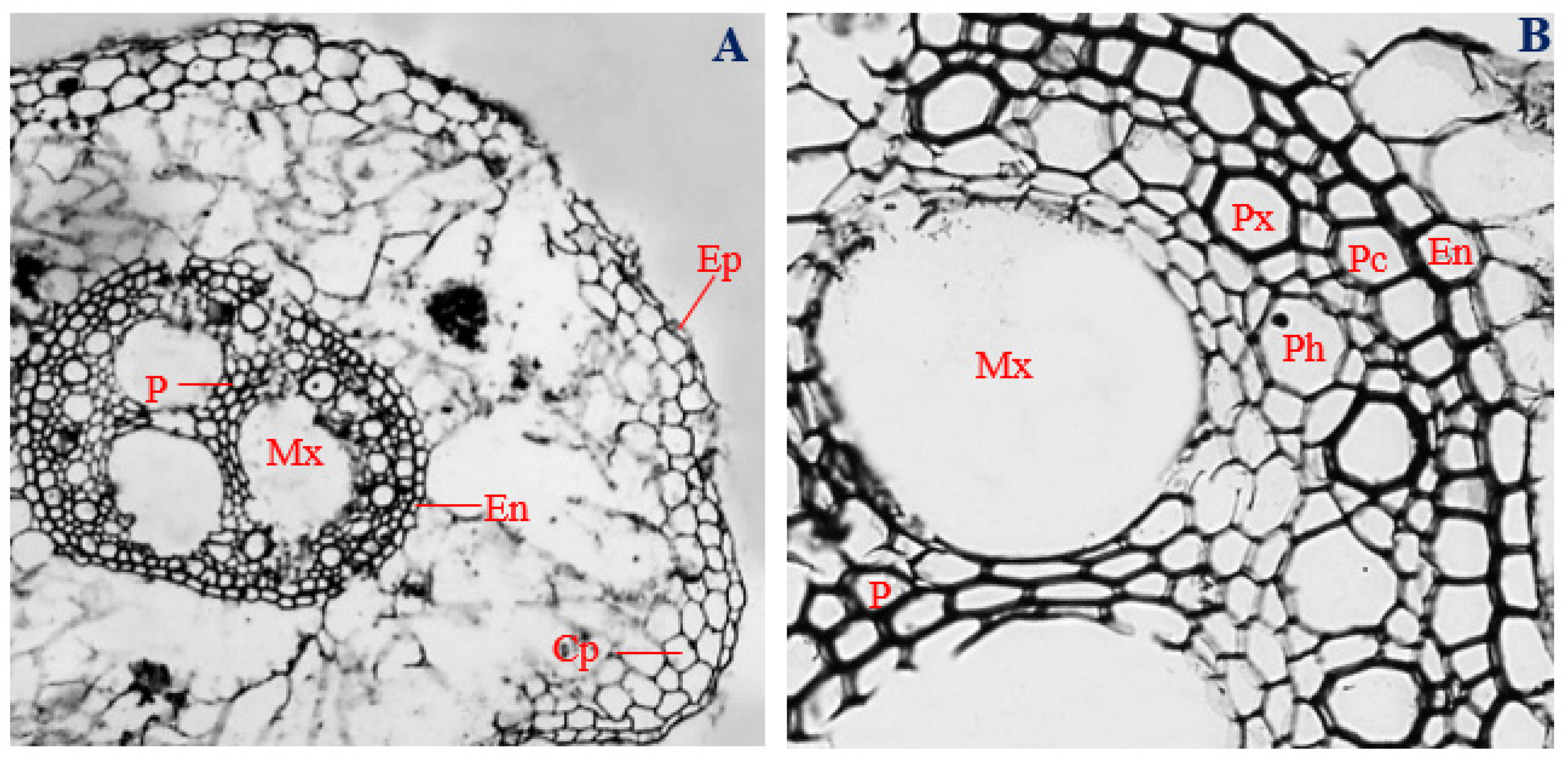This set of two black and white microscope images, each labeled in the top right corner with 'A' and 'B' respectively, appears to show a cross-sectional view of a cellular structure resembling a network of bubbles. The first image, labeled A, presents a roughly circular mass with several concentric circles and radial labels in red text. Key labeled components within this image include: the center marked 'MX', adjacent circles labeled 'P', 'EN', 'CP', and the outer border marked 'EP'. 

Image B provides a closer, more detailed view of the central portion of image A, focusing primarily on 'MX'. It identifies additional cellular components in closer proximity: 'P', 'PX', 'PH' (with a dark dot in its center), 'PC', and 'EN'. Together, these labels likely represent abbreviations for different parts of the cellular structure, offering a detailed scientific visualization of the specimen.